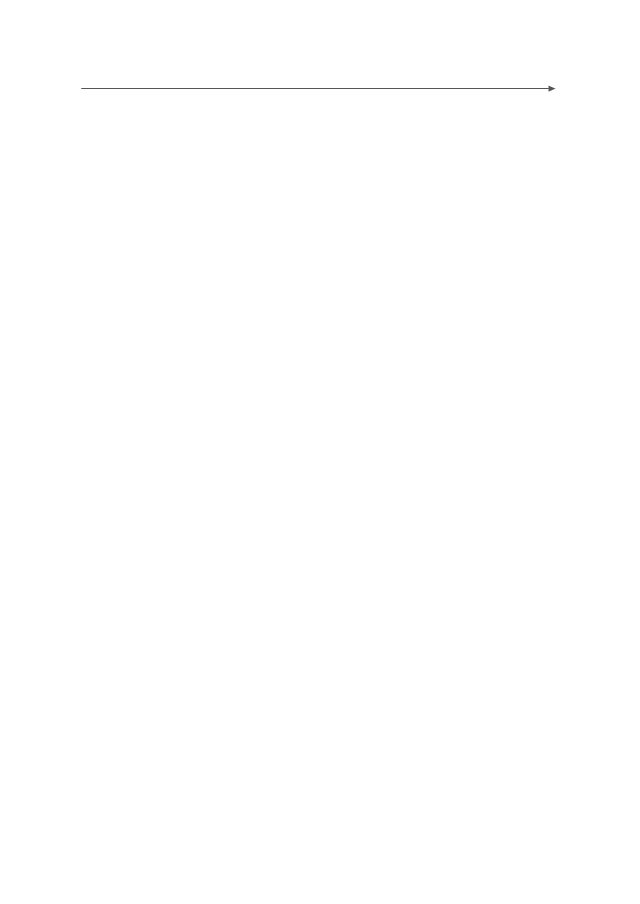The image appears almost entirely blank, as if it hasn't fully loaded or is intentionally minimalistic. There are no borders, shapes, or textual elements. The stark expanse is occasionally interrupted by a very thin, dark gray, almost black, arrow stretching across the top. The arrow spans the full width of the image, drawing attention with its subtlety. 

The arrow is unusually delicate, requiring close inspection to discern its path. At the far right end, a small, equally thin triangle indicates the arrow's direction, pointing to the right and suggesting a focus or movement in that direction. The minimalism of the arrow might imply an understated emphasis or a discreet indication towards something significant off-frame. 

Overall, the image merges with the background seamlessly, enhancing its sparse and nearly invisible nature. It demands careful observation, as the arrow's delicate presence could easily be overlooked without scrutiny. The simplicity of the image underscores a unique visual narrative, subtly nudging the viewer towards the right.